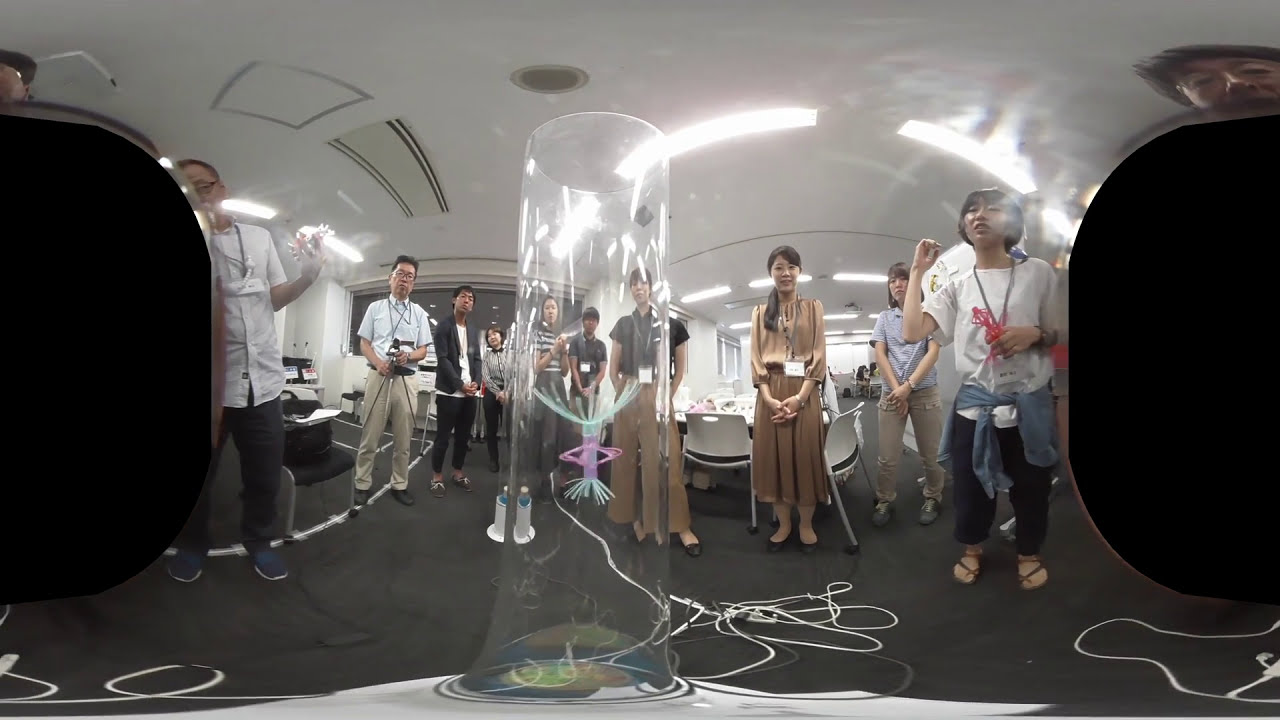In this image, we see a group of approximately 10 or 11 people gathered in a room, seemingly engaged in a presentation or demonstration. The participants, mostly Asian men and women, are standing on a gray carpeted floor with white power cords scattered around. The room has white walls and a white ceiling illuminated by ceiling lights. 

In the foreground, dominating the scene, is a tall, clear acrylic cylindrical tube with several wires coming from it. Inside this tube is a fascinating object, featuring stringy elements with light teal green and purple tones, floating and suspended mid-air, which adds a sense of intrigue. On the left and right sides of the image, there are black, rounded shapes, potentially caused by a distorted, curved camera lens.

Among the onlookers, one man with glasses in a white shirt is intently examining a black square device. Another notable figure is a woman with a white t-shirt, a jacket tied around her waist, and sandals. Another woman, wearing a light purple shirt, stands nearby. The crowd appears to be engaged, some smiling, and one even cheering, adding a lively atmosphere to the scene. The background features a white table with white chairs.

The overall color scheme includes predominant shades of white, brown, and tan, with splashes of pink, green, and blue, creating a somewhat clinical and focused environment.